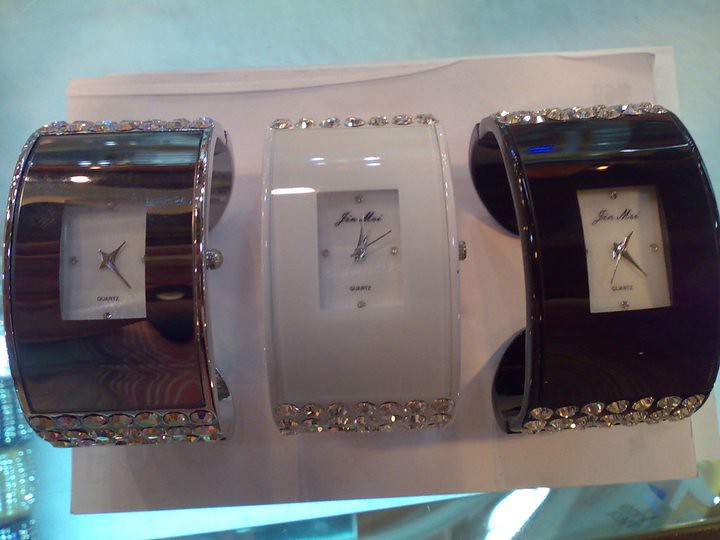The image showcases three elegant women's wristwatches displayed on a white, rectangular sheet of paper atop a see-through glass display case illuminated from below by a subtle blue light. Each watch resembles a sophisticated bracelet or bangle, featuring a sleek, wide band adorned with small crystal studs that may or may not be real diamond. The watches come in three distinct colors: the one on the left is brown, the center one is white, and the one on the right is black. The timepieces themselves are beautifully crafted, with silver and possibly gold detailing, and all feature the label 'quartz.' Each watch displays only the hour and minute hands, lacking a second hand.